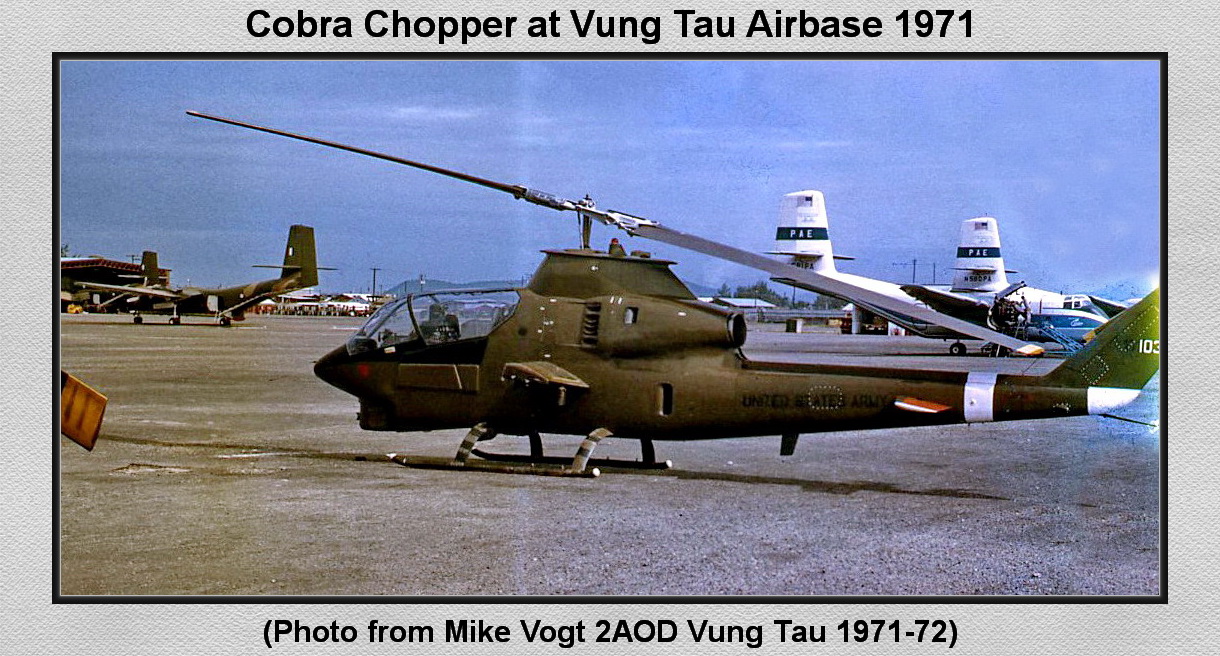This vintage photograph, taken at Vung Tau Airbase in 1971, depicts a dark green United States Army helicopter, known as a Cobra Chopper. The helicopter, identifiable by its tail number 103 and "United States Army" emblazoned on its side, sits on the gray concrete ground of the airbase, its two blades positioned diagonally. The background features blue skies and other pieces of military equipment, including a large white aircraft with two wings. The photo is bordered in light gray with a header that reads "Cobra Chopper at Vung Tau Airbase 1971" and a footer in parentheses stating "photo from Mike Vogt to AOD Vung Tau 1971-72." The cockpit of the chopper is notably empty, emphasizing its stationary state.